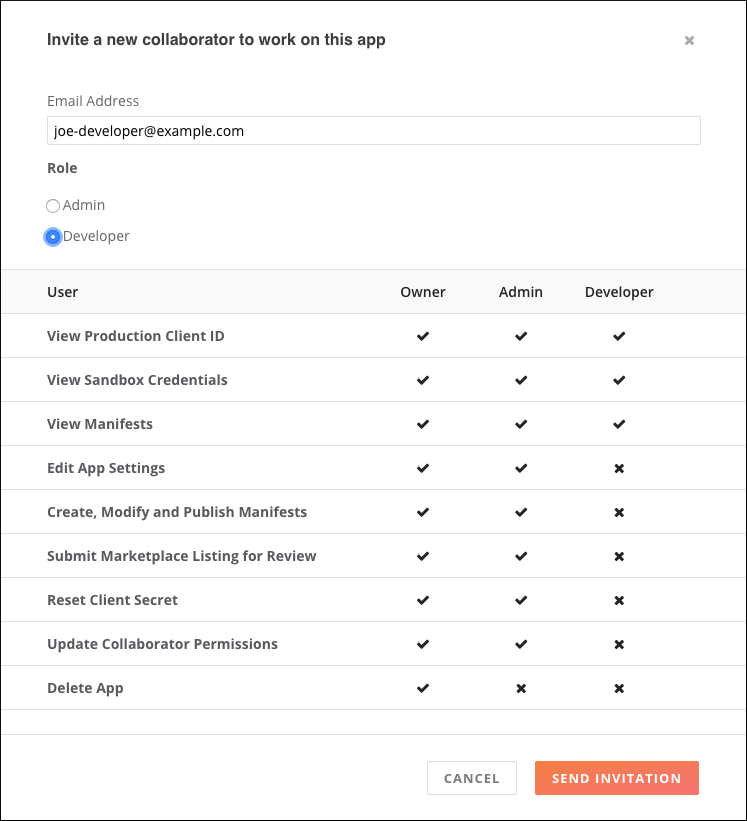A detailed caption for the described image could be:

The image displays a form with a white rectangle bordered by a black line on all four sides. At the top of the form, bold black text reads, "Invite a new collaborator to work on this app." Below this header, there is a field labeled "Email Address" followed by a text box containing the example email address "joe-developer@example.com."

Beneath the email address field, the label "Role" is positioned next to two radio buttons labeled "Admin" and "Developer," with the "Developer" option selected and highlighted in blue. The selected role reveals specific permissions listed vertically below, starting with "User," followed by a series of options: "View production client ID," "View sandbox credentials," "View manifest," "Edit app settings," "Create, modify, and publish manifest," "Submit marketplace listing for review," "Reset client secret," "Update collaborator permission," and "Delete apps."

To the right of these permissions, three columns are labeled "Owner," "Admin," and "Developer," which likely indicate the access level options for the listed permissions. At the bottom of the form, there are two buttons—"Cancel" on the left and "Send Invitation" on the right.